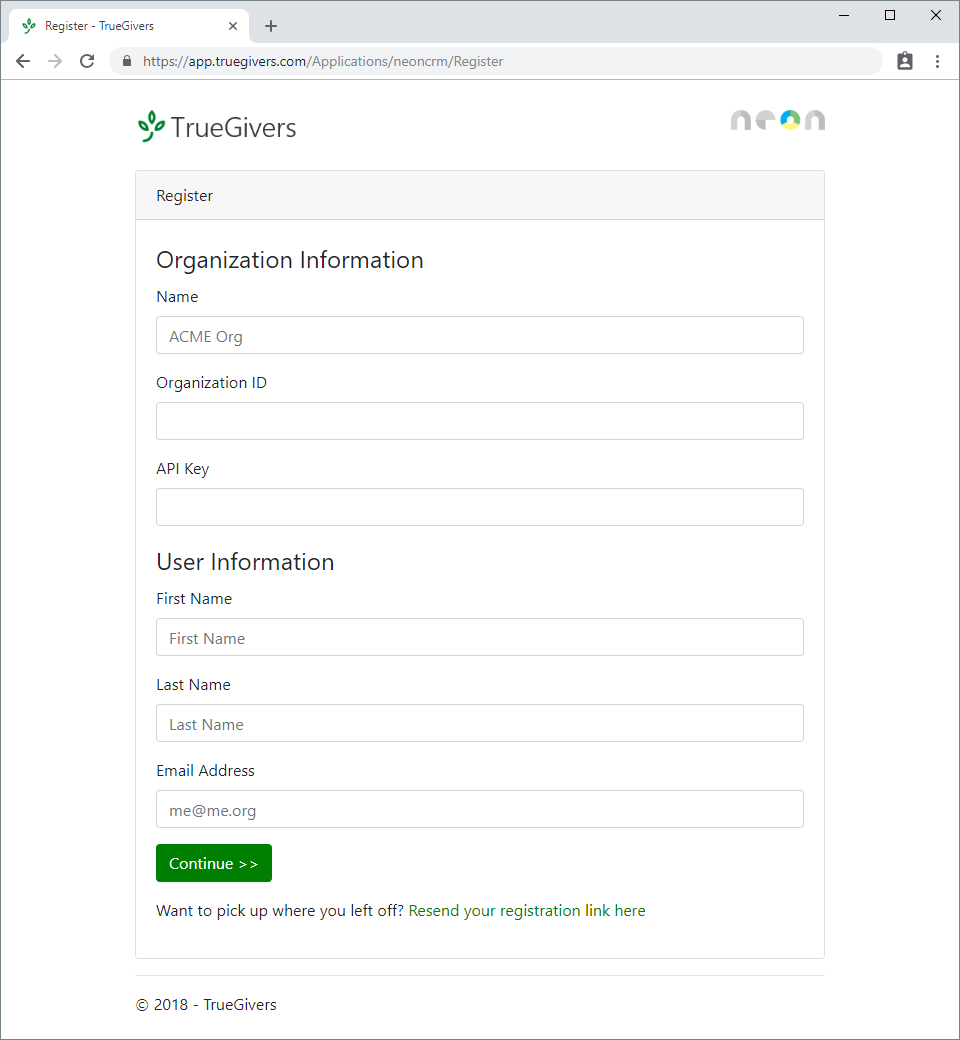This image is a screenshot of a registration page from the website app.truegivers.com. At the top of the page, the logo "TrueGivers" is prominently displayed, accompanied by a graphic of a small branch with three leaves. Beneath the logo, the text "register" is featured.

The page is divided into sections for "Organization Information" and "User Information." Within the "Organization Information" section, there is a label for "Name" with the example "acme.org" typed in the corresponding input box. The "Organization ID" field is present but left blank. Below that is a field labeled "API Key," which is also blank.

The "User Information" section includes fields for "First Name," "Last Name," and "Email Address." The input boxes for "First Name" and "Last Name" both contain placeholder text that says "first name" and "last name," respectively. The "Email Address" input box is empty, waiting for user input.

At the bottom of the registration form, there's a green button labeled "Continue." Below this button, a link is provided with the text "Want to pick up where you left off? Resend your registration link here," indicating users can click to resend the registration link if needed.

Finally, the footer of the page contains the text "Copyright 2018 TrueGivers."

This detailed description provides a clear representation of the elements and layout of the registration page.